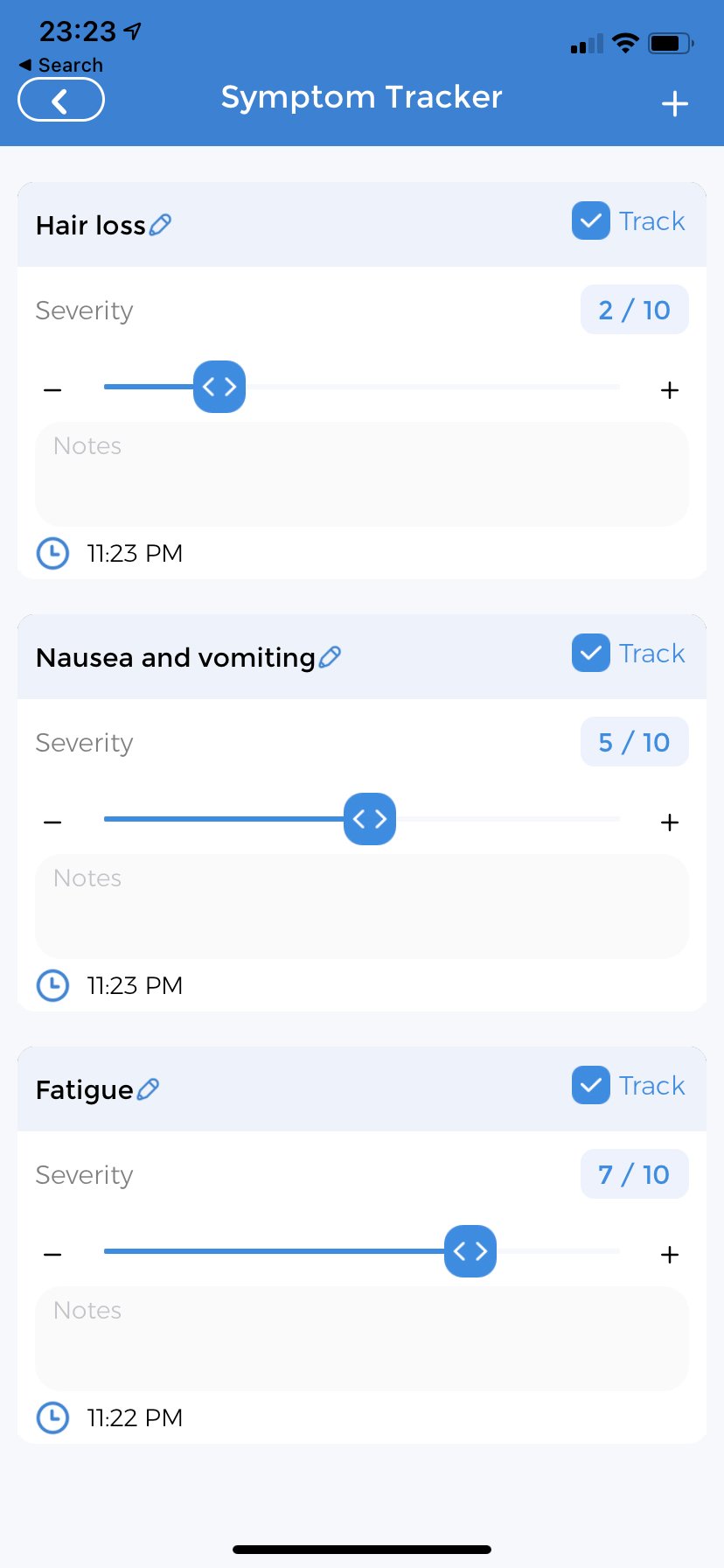This detailed caption provides a comprehensive overview of a cell phone screen displaying a symptom tracker app:

---

The image showcases a cell phone screen with a symptom tracker app displayed. At the very top left, the time reads "23:23," followed by a small word "Search" and a left-facing arrow below it. Moving to the right, a connection icon shows two out of four bars filled in black. Further right, a Wi-Fi icon is situated next, followed by a battery icon indicating approximately 70-80% charge.

The header of the app has a blue background. "Symptom Tracker" is prominently displayed in white text, complemented by a white plus sign to its right.

The main part of the interface features alternating small gray rectangles for symptom names against a predominantly white background:

1. **Hair Loss (2/10)**:
   - Track button with a blue checkmark box.
   - Severity: 2 out of 10.
   - Notes timestamped at 11:23 PM.

2. **Nausea and Vomiting (5/10)**:
   - Track button.
   - Severity: 5 out of 10.
   - Notes timestamped at 11:23 PM.

3. **Fatigue (7/10)**:
   - Track button with a blue checkmark box.
   - Severity: 7 out of 10 (highlighted in blue with a gray background).
   - Notes timestamped at 11:22 PM with a blue clock icon to its left akin to the other symptoms.

The bottom of the screen features a black horizontal bar, completing the detailed view of the symptom tracker app from top to bottom.